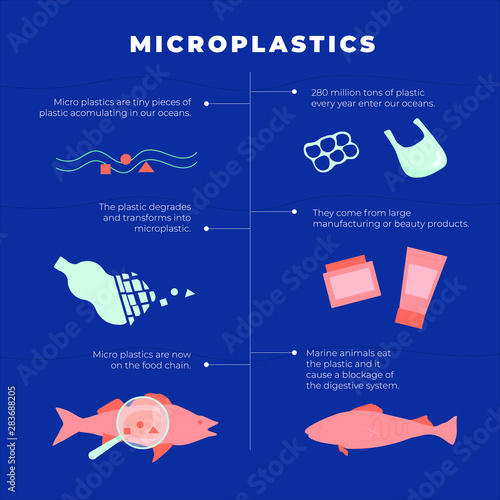The image is a detailed infographic with a dark blue background. At the top, in bold white capitalized letters, it reads "MICROPLASTICS." The infographic illustrates how microplastics accumulate and impact marine life.

Starting from the top left, the caption explains that microplastics are tiny pieces of plastic accumulating in our oceans, accompanied by an image of wavy water and plastics. On the right, it states that 280 million tons of plastic enter our oceans every year, depicted by a plastic six-pack holder and a plastic bag.

Moving downwards, the infographic describes how these plastics degrade and transform into microplastics, showing a plastic bottle breaking down. It also notes that these microplastics originate from large manufacturing and beauty products, with illustrations of a red tube and jar of beauty products.

At the bottom left, the infographic warns that microplastics are now in the food chain, with a fish image magnified to highlight plastics inside its stomach. On the right, it shows marine animals eating the plastics, leading to digestive blockages, illustrated by a red-colored fish suffering from ingestion issues.

Overall, the infographic provides a comprehensive and visually engaging explanation of the dangers of microplastics in our oceans.